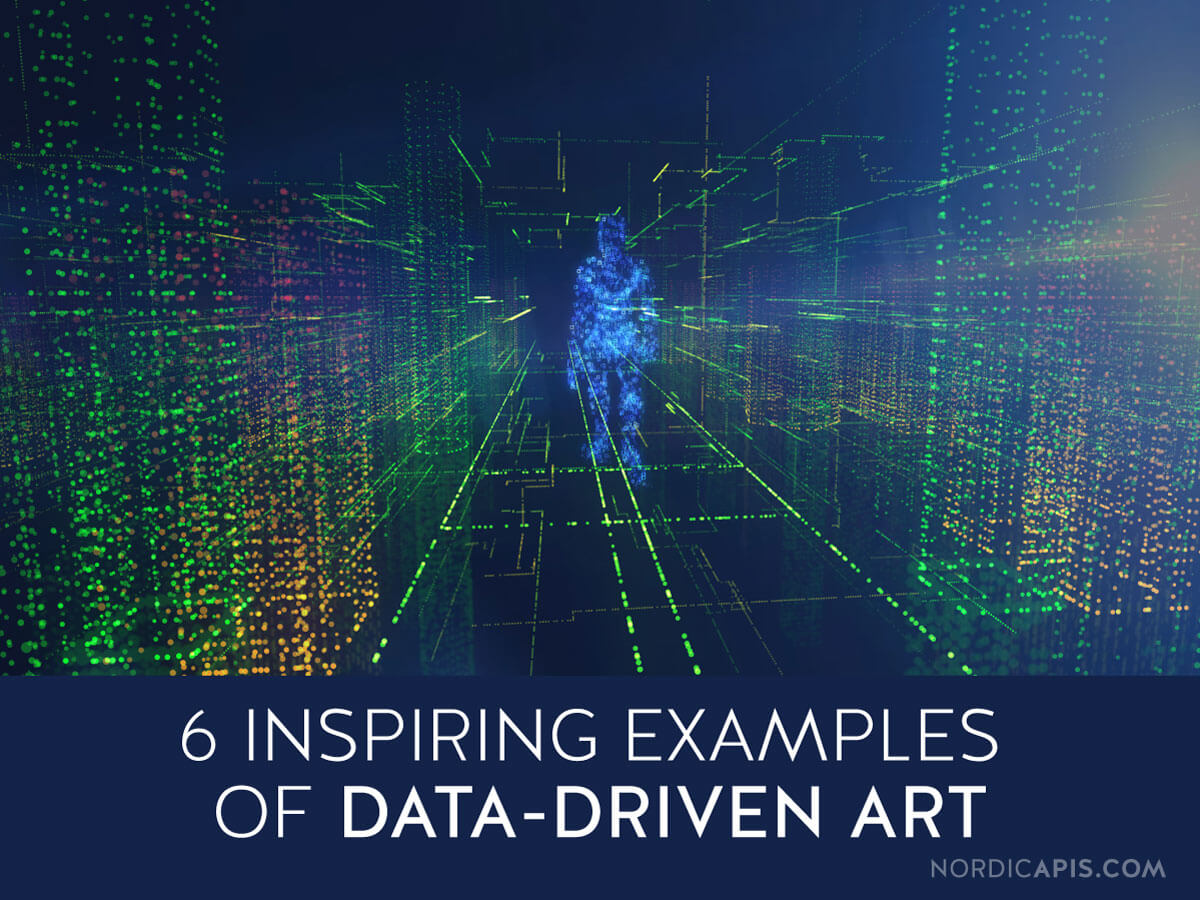The image is a detailed, futuristic representation of cyberspace, highlighting data-driven art. A dark blue border at the bottom contains white text that reads, "Six inspiring examples of data-driven art. Nordicapis.com." Above this border, a series of green dots and moving lights create an electronic, almost digital environment. The scene is dominated by green light pillars that outline a central hallway, dotted with green lights. At the center of the image, a figure made of blue, electrical static appears to be walking away from the viewer, adding to the pixelated and digital aesthetic. Orange lights, resembling server towers, are positioned along the edges, further enhancing the sense of a virtual space. The overall composition conveys a high-tech, cybernetic world.